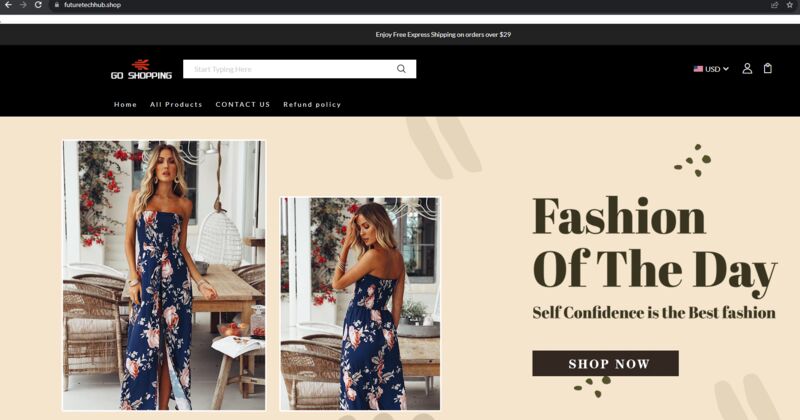A screenshot taken from a website showcases a variety of elements. At the very top, there is a thin black bar. On the left side of this bar, there is a white arrow pointing left, a gray arrow pointing left, a gray arrow pointing right, and a blue and white refresh icon. Adjacent to these icons is a website link in white text, which is too small to read.

Beneath this bar, at the center, is a section with white text on a black background, which is also too small to read. Below this, spanning from the left to the right, is a red logo at the top and the text "Go Shopping" in white below it. Next to this is a white search bar. On the right-hand side of this section, there is an icon of the U.S. flag, followed by the text "USD", a picture of a person, and a shopping bag icon.

Following this, under the "Go Shopping" text, there are four clickable boxes labeled "Home", "All Products", "Contact Us", and "Refund Online".

The main content area features a gray background with an image of a white woman wearing a stylish white and blue sundress. She has fake blonde hair. In one picture, she is looking directly at the camera, while in another, she has her back turned but is glancing over her shoulder.

On the right side of the image, there is black text that reads, "Fashion of the Day: Self-confidence is the best fashion." Below this text is a black box with white text that says, "Shop Now."

The caption concludes with a note of gratitude to "Matt and his team," indicating this might be the last screenshot provided for a while.

This enhanced description covers all the elements described in the voice caption in a structured and detailed manner.